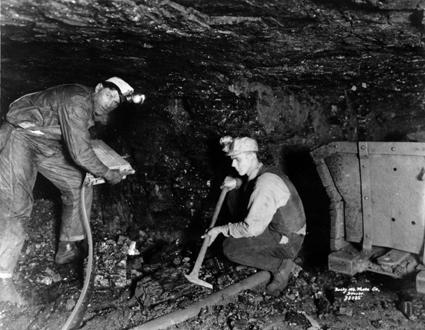This black and white photograph captures a narrow, low-ceilinged underground coal mine scene with two men engaged in labor. On the left side of the image, a tall miner dressed in long sleeves and pants is in a lunge position, with his left knee forward and right leg straight. He is bent at the waist and clutching a rectangular, cabled object, which could be machinery or a mining tool, and he has a hard hat with a light affixed to it, illuminating his surroundings as he gazes towards the camera. To his right, another miner is crouched down low with bent knees, almost touching the ground. This second miner is also in long sleeves and pants, complemented by a vest and boots. He wields a long-handled instrument resembling a pickaxe, implying he is about to work the ground in front of him. Both men exhibit the grime typical of mine work. Positioned beside the crouched miner is a light gray ore cart, suggesting they might be digging out ore and transporting it via this cart. The claustrophobic setting with dark walls enhances the perception that they are deep within a coal mine.